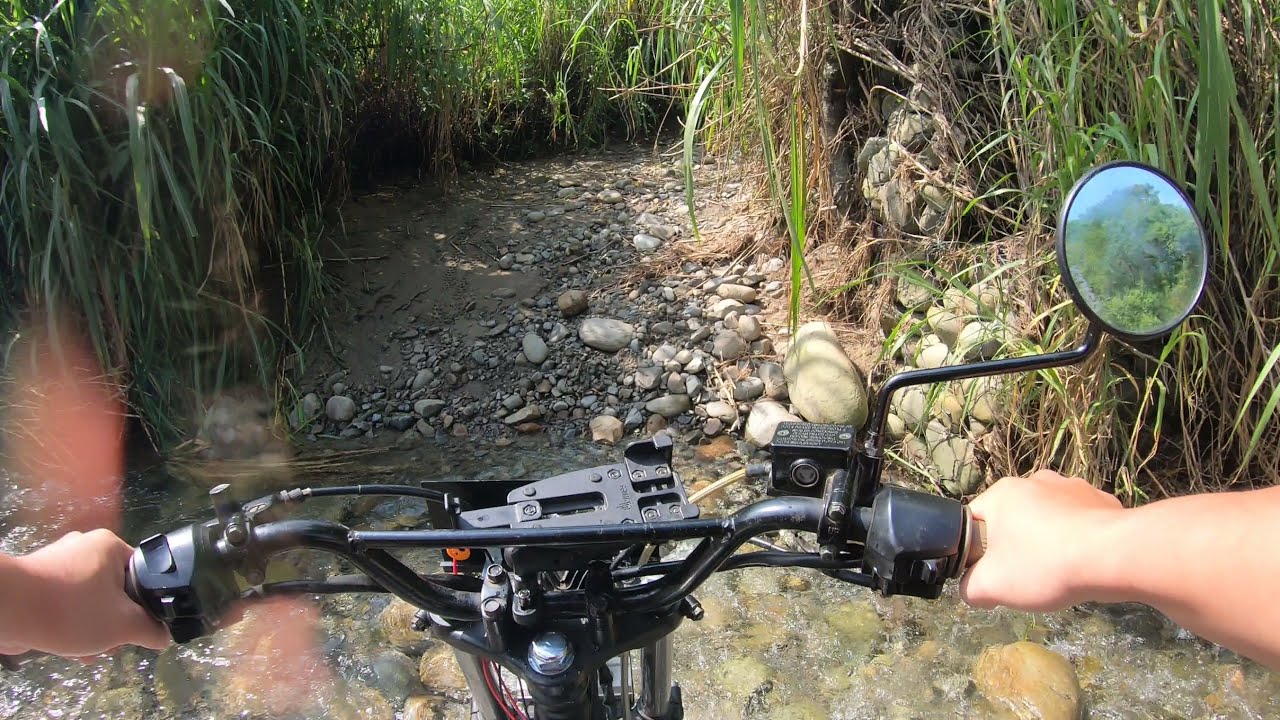This color exterior daylight photograph captures the perspective of a rider navigating a black, advanced-looking motorbike or heavy-duty mountain bike, possibly equipped with electronic elements, over a shallow, rocky stream. The viewpoint is first-person, looking down over the complex mechanical structure of the handlebars, which include bright silver metal components and a large circular side mirror on the right side, reflecting lush green trees. The rider's light-skinned arms and hands firmly grip the handles. Beneath the bike, clear, flowing water reveals an array of stones. Emerging from the stream, the path transitions into a gray dirt and rock trail lined with tall green grasses, reminiscent of a cornfield, and curves away to the right, enveloped by vibrant vegetation.